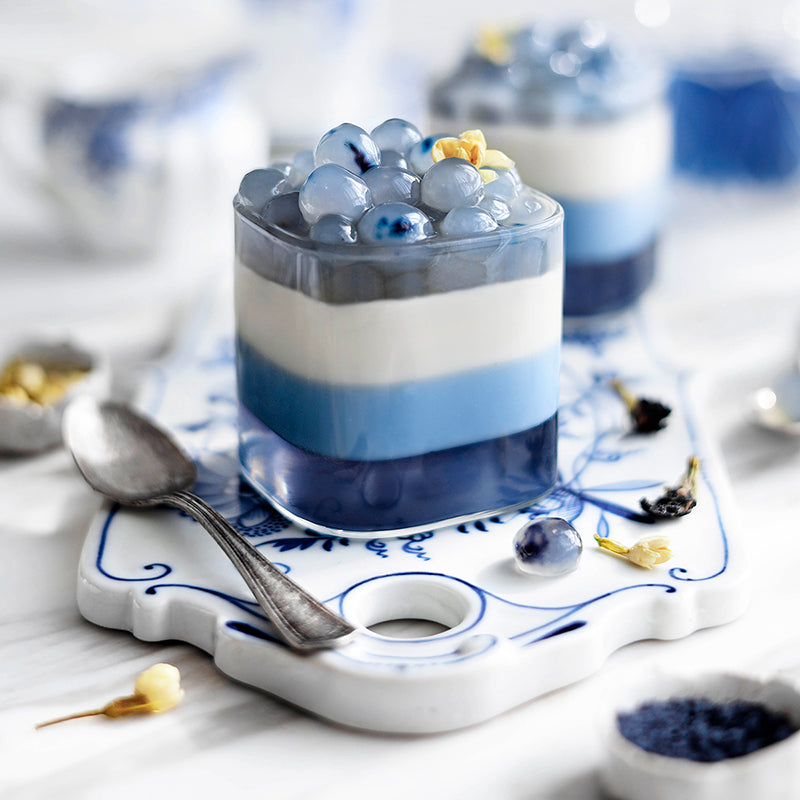The image depicts a visually stunning butterfly pea dessert served in a square glass cup. The dessert features distinct layers: the bottom layer is dark blue, followed by a light blue layer, a middle white layer, and a top adorned with small, globular shapes which could be sago crystals or boba pearls. Additionally, a bright yellow flower is elegantly placed on top, enhancing the overall presentation. The dessert sits on a white cutting board, which is decorated with scattered yellow and dark blue flowers as well as blue powder, adding aesthetic appeal. To the left of the cup, there is a silver spoon, while to the bottom right, a small bell is visible. Another drink can be seen in the background, further complementing the dessert setting.